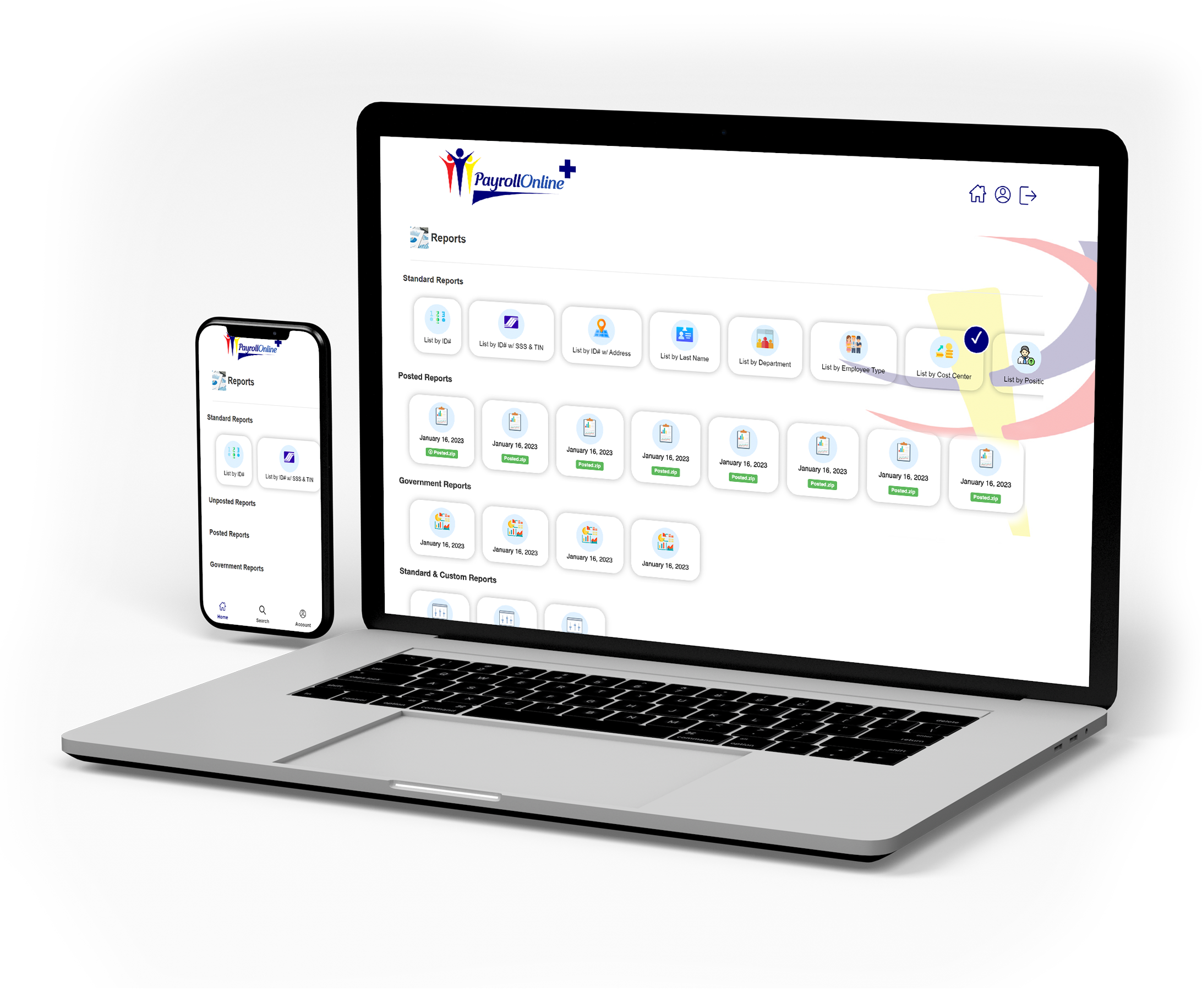In the image, there's a screenshot from a company called Payroll Online, showcasing its interface on both a laptop and a phone. The laptop screen is slightly off-center and tilted to the left, but the content is still partially visible. At the top of the screen, set against a white background, are icons of people in various colors—red, purple, and yellow. The main heading reads "Payroll Online" featuring a large blue plus symbol next to it. Beneath this, the word "Reports" is clearly displayed, followed by a horizontal line. The section labeled "Standard Reports" lists eight items, though the details are hard to decipher due to the screen's angle.

Further down, another section appears with a similar layout, containing eight listings under a second category of reports. Below this, there's a category labeled "Government Reports" with four items. The final visible section is labeled "Standard and something Reports," listing three items. The bottom part of the screen bears the name "Payroll Online" again, indicating the service's main operations.

The phone version of Payroll Online is also shown, featuring a more condensed layout with less information displayed compared to the laptop version. This service appears to cater to small businesses, providing a streamlined solution for payroll management. Instead of hiring a dedicated payroll employee, businesses can utilize Payroll Online to handle their payroll needs efficiently.